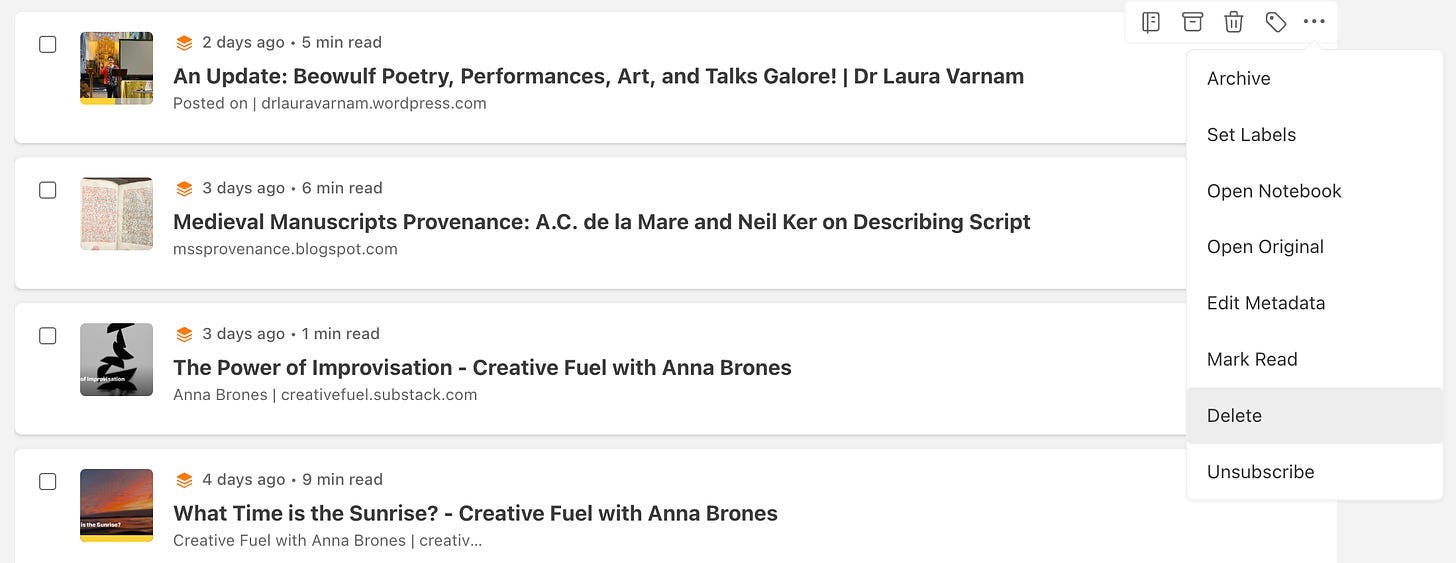This image is a screenshot taken from a literature-focused website. The details of the website's name have been cropped out from the top of the image. At the top of the image, there is an entry labeled "Two days ago" with a "five-minute read" tag. This entry is titled "An Update: Bail with Poetry Performances, Art, and Talks Galore" by Dr. Laura Varnum, accompanied by her contact information from her WordPress account.

Below this is another entry labeled "Three days ago" with a "six-minute read" tag. The title for this entry is "Medieval Manuscripts: Provenance AC de la Mayor and Neil Kerr on Describing Script."

Further down, there is an entry labeled "Three days ago" with a "one-minute read" tag. This one is titled "The Power of Improvisation: Creative Fuel" by Anna Brown.

Finally, at the bottom, there is another entry related to Anna Brown, titled "What Time is the Sunrise? Creative Fun with Anna Brown." Each entry succinctly captures various aspects of literature, from poetry and medieval manuscripts to creativity and improvisation.